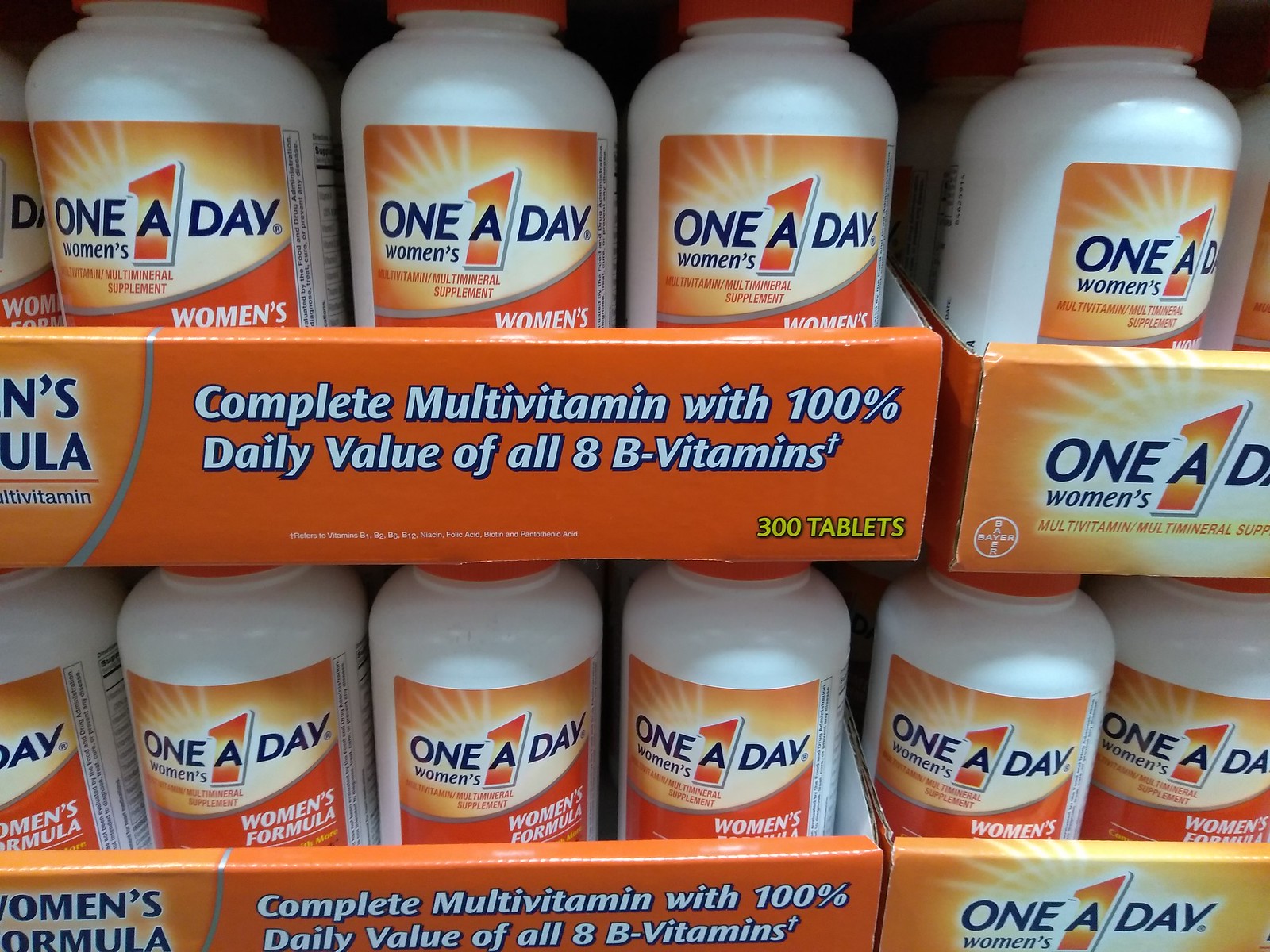The image showcases multiple large, white bottles of One-A-Day Women's multivitamins, each featuring an orange cap. The photograph seemingly captures a store display, as several identical bottles are grouped together. The label on each bottle prominently reads "One-A-Day Women's," along with various other details in smaller text that are not clearly legible. These vitamin bottles are neatly arranged within cardboard boxes. The front of the box is designed with an orange and white gradient on the left side, transitioning to a darker orange on the right. In white text against the orange background, it states, "Complete Multivitamin with 100% Daily Value of all 8 B Vitamins" and highlights that each bottle contains 300 tablets. Each visible box appears to contain four bottles of vitamins, though it is unclear if there are additional bottles behind those in the front. Altogether, four boxes can be seen in the image.